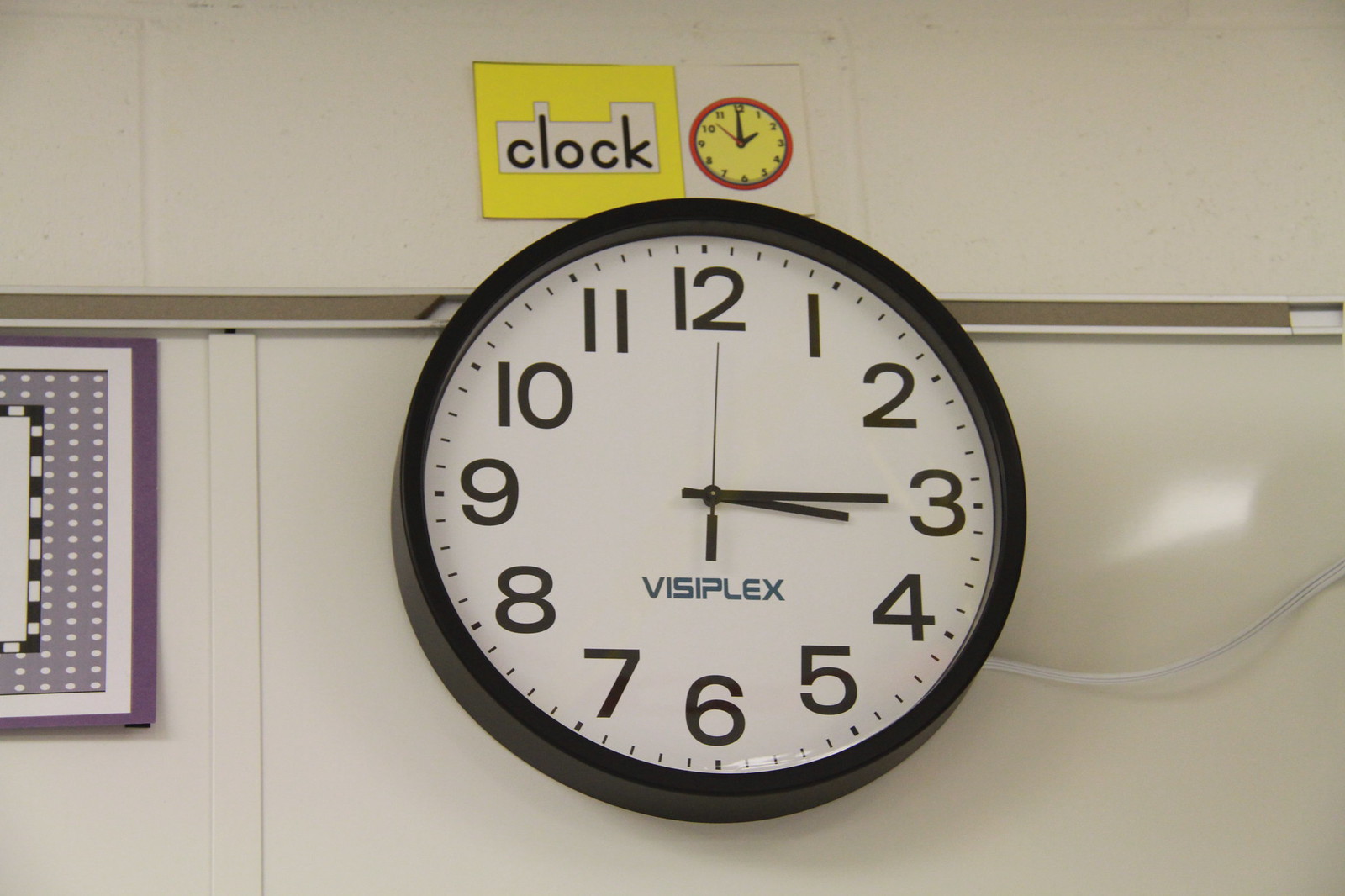A round-faced wall clock with a sleek black body hangs prominently on a stark white wall. The clock's clean, white face houses precise, dark hour markers and hands, complemented by the name "Vesiclex" written in a distinctive blue font beneath the clock's center. Adjacent to this, an unobtrusive white electric cord trails from the back of the clock and extends to the edge of the image. Above the clock, a piece of yellow and white cardboard displays the word "Clock" in bold black letters, alongside an image of a vibrant red and yellow clock, adding a playful touch to the overall presentation.